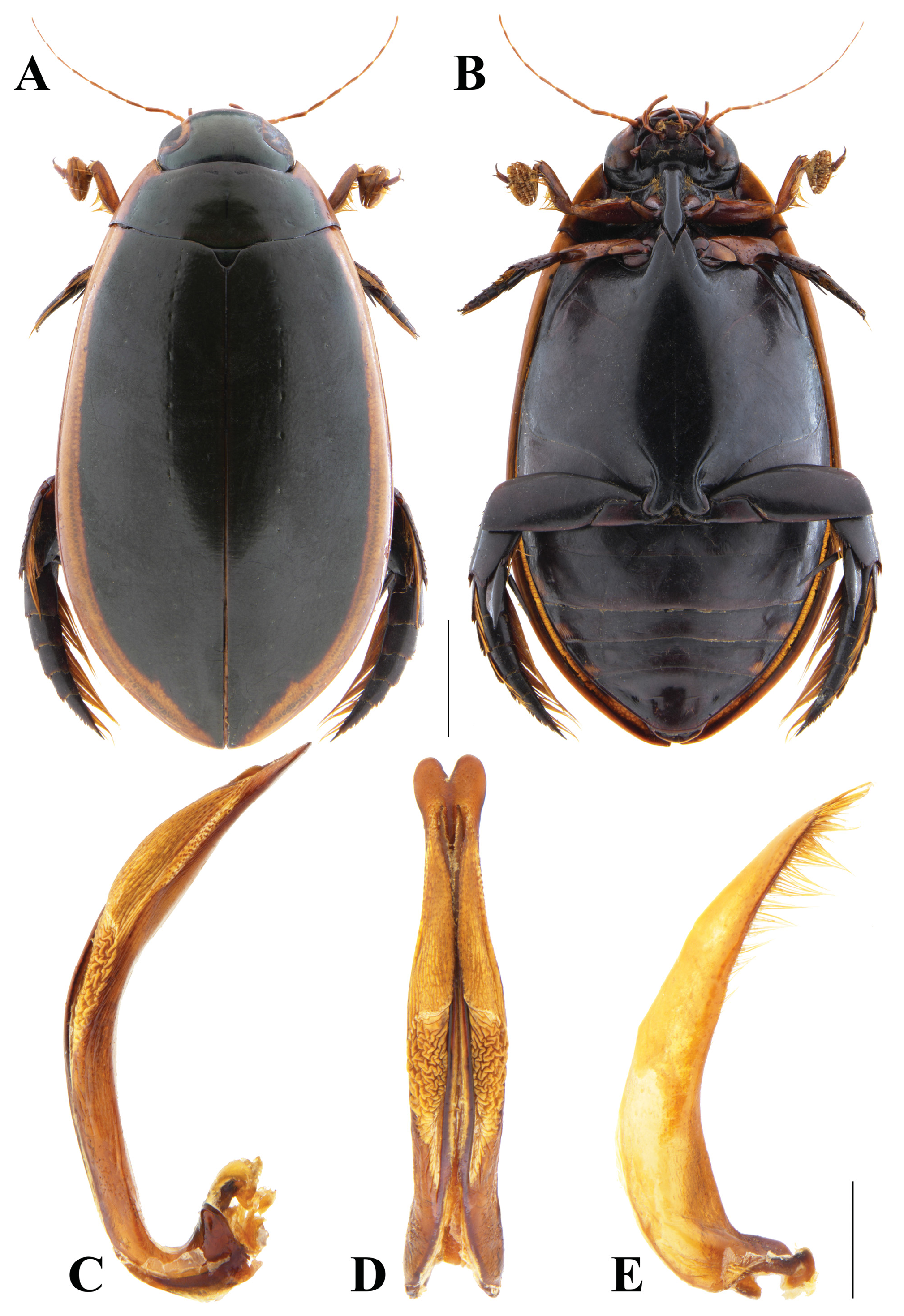The image consists of a detailed scientific depiction featuring five labeled photographs of a beetle-like insect, likely a cockroach. Photograph A presents the dorsal view (top) of the insect, showing its black back with brown edges. Photograph B illustrates the ventral view (underside) of the roach. Photograph C displays one of the insect’s legs, appearing goldish brown. Photograph D depicts an internal part of the insect, possibly an intestine. Photograph E shows another leg or possibly an antenna. The insect has two prominent antennae, multiple legs (six), and appears to have distinct brown and black coloring not native to America. The photographs are precise and realistic, suitable for educational or scientific purposes.